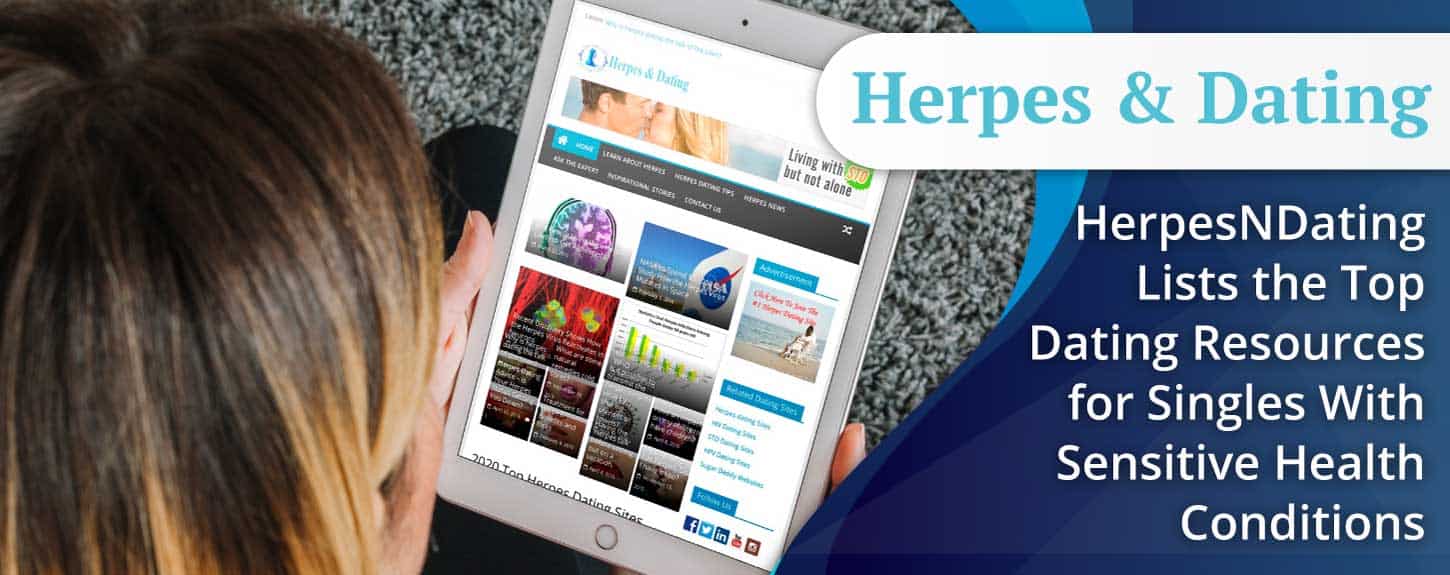The image is centered around resources for dating with herpes. At the top, there is a white pill-shaped box with the words "Herpes & Dating" written in blue text. This phrase is repeated below in white letters, with an "N" in between "herpes" and "dating." 

The background is predominantly blue, featuring a wave-like design that starts in the center and curves upward towards the right. On one side of the image, there is a woman holding a tablet that displays text related to herpes and dating, emphasizing that living with an STD does not mean being alone. 

The woman, who has light skin and brown hair accented with blonde streaks, is depicted against a backdrop that includes a rug. The multitude of images on the tablet illustrates the various resources and support available for singles with sensitive health conditions.